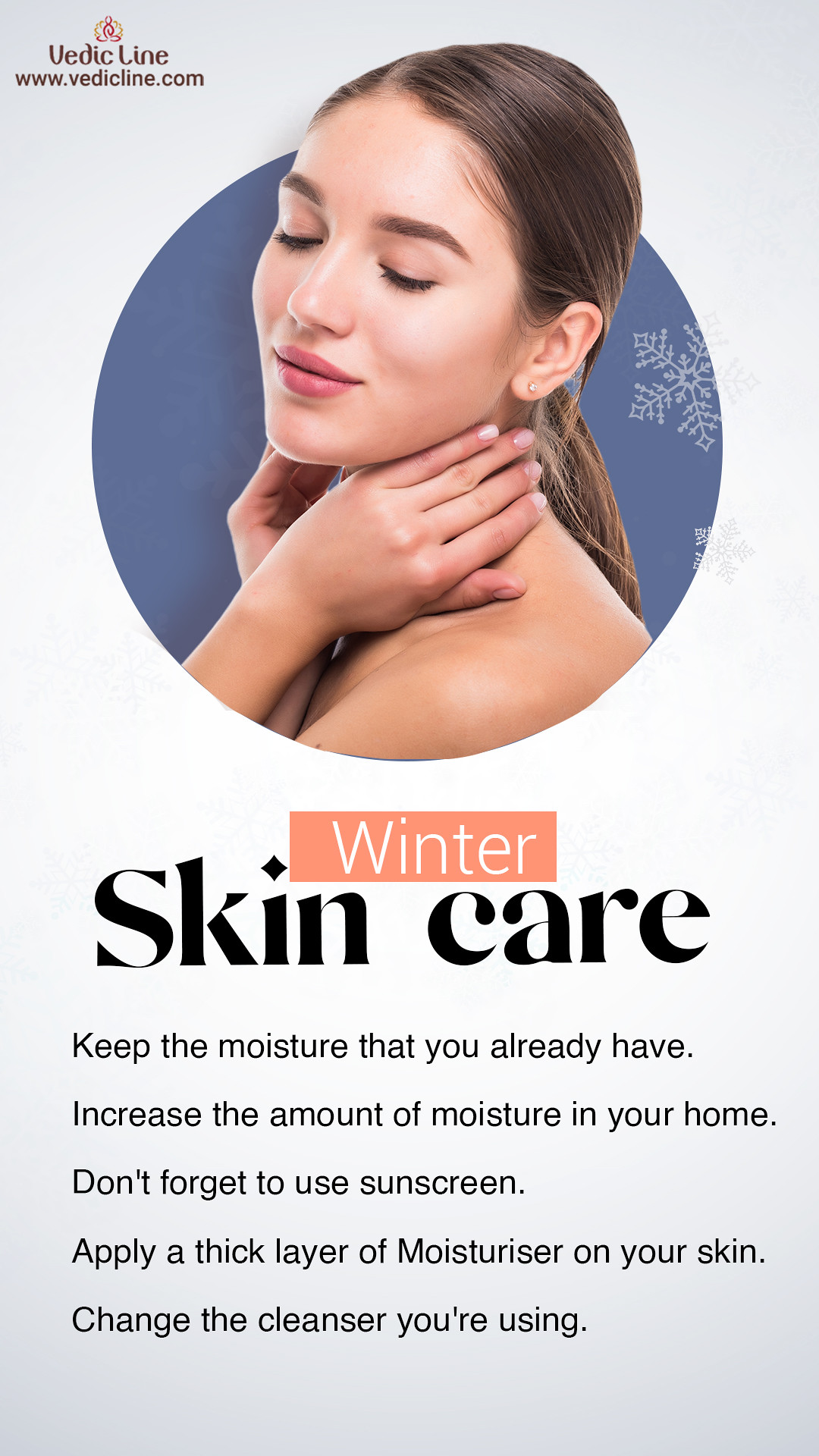The image portrays a detailed advertisement for winter skincare products from the brand VedicLime. The central focus is a young woman seen from the shoulders up, with her dark hair pulled back in a ponytail. She appears relaxed, with her eyes closed and a gentle smile, as she rubs her neck, possibly applying skincare product. The ad features a soft, muted blue background with a subtle snowflake-star design on the right side, enhancing the winter theme. The text beneath the model provides detailed winter skincare tips, emphasizing the importance of retaining moisture, increasing home humidity, using sunscreen, applying thick moisturizer, and changing cleansers. At the top left corner, the brand's logo, VedicLime, along with their website, VedicLime.com, is prominently displayed. The text below the model is highlighted on an orange backdrop, with larger text reading "Winter Skin Care" followed by additional information in smaller black font.